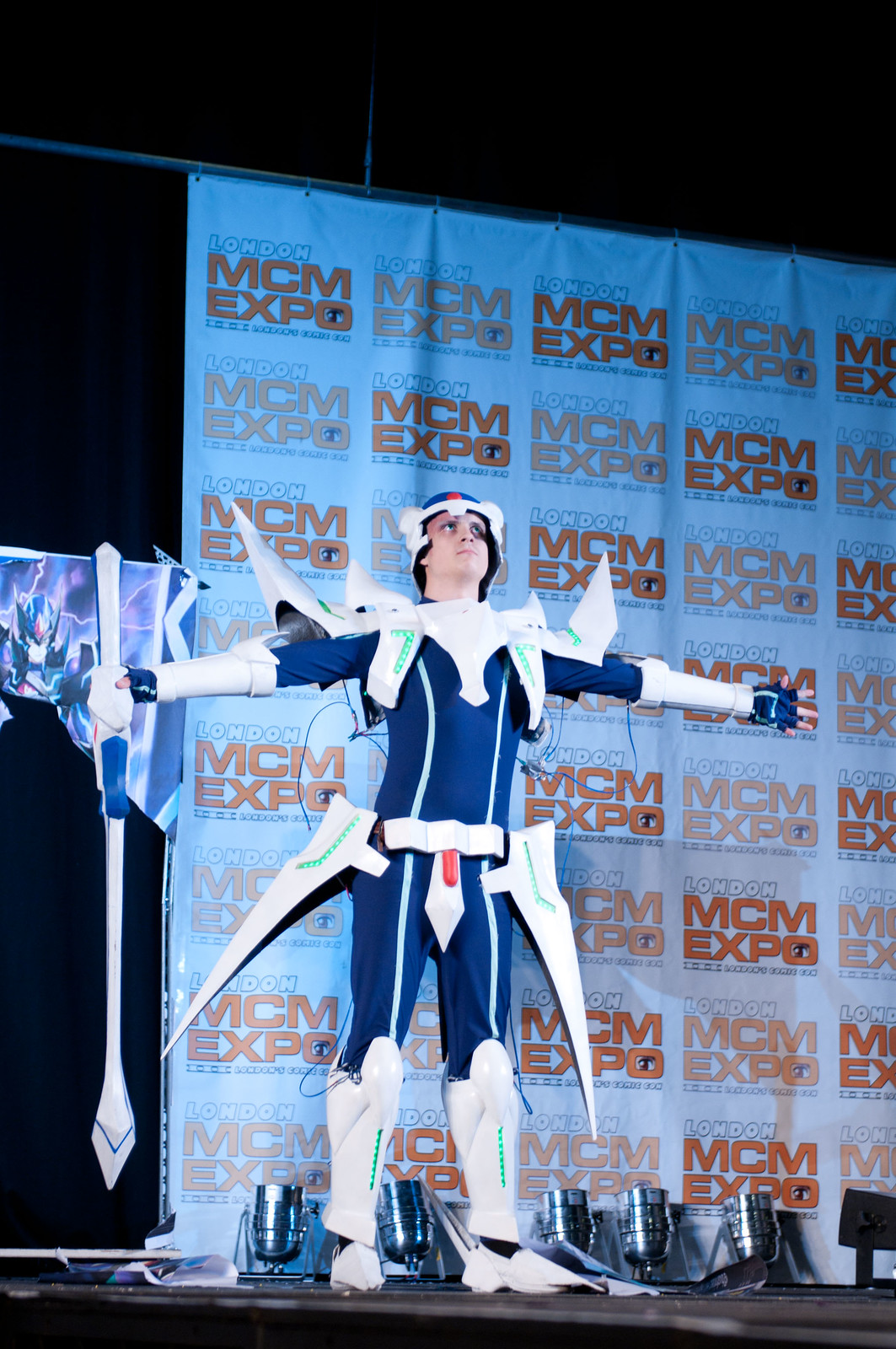A young male cosplayer is captured on stage at the London MCM Expo, striking a dramatic pose with outstretched arms and gazing upwards. He is dressed in a figure-hugging blue costume with darker blue and whitish stripes. His outfit features elaborate, plastic-looking white body armor, including muscular and pointed shin covers, knee-high boots, and a series of pointed elements around his hips and shoulders that extend upwards. The costume also includes green LED lights that add an ethereal glow and are connected by visible wires. His accessories include a blue helmet with white sections around the ears and a distinctive white sword held in his left hand. The background displays a large tarpaulin backdrop with a repeating "London MCM Expo" logo, illuminated by spotlights that accentuate the scene.